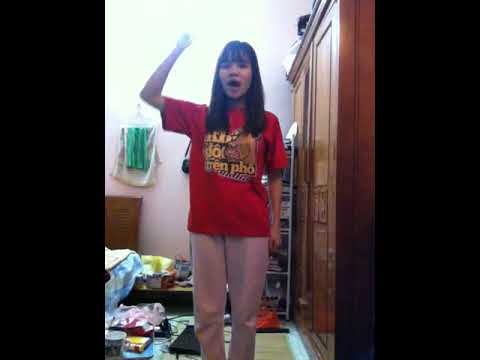A young woman of likely Asian descent is standing in what appears to be her cluttered bedroom, a brightly lit room with white-pink walls. Her long black hair, with straight bangs, frames her face. She wears a red t-shirt adorned with a yellow logo and light pink sweatpants. Her left hand is raised in the air, possibly making a fist, and her mouth is open as if she’s speaking. To her right is a tall, shiny brown wooden armoire, while to her left is a mattress with a wooden headboard. Behind her is a white-framed shelving unit and various items strewn across the floor, including clothes, books, and possibly a mug. Towels hang on the wall alongside the disarray of personal belongings, creating a scene of casual domesticity.